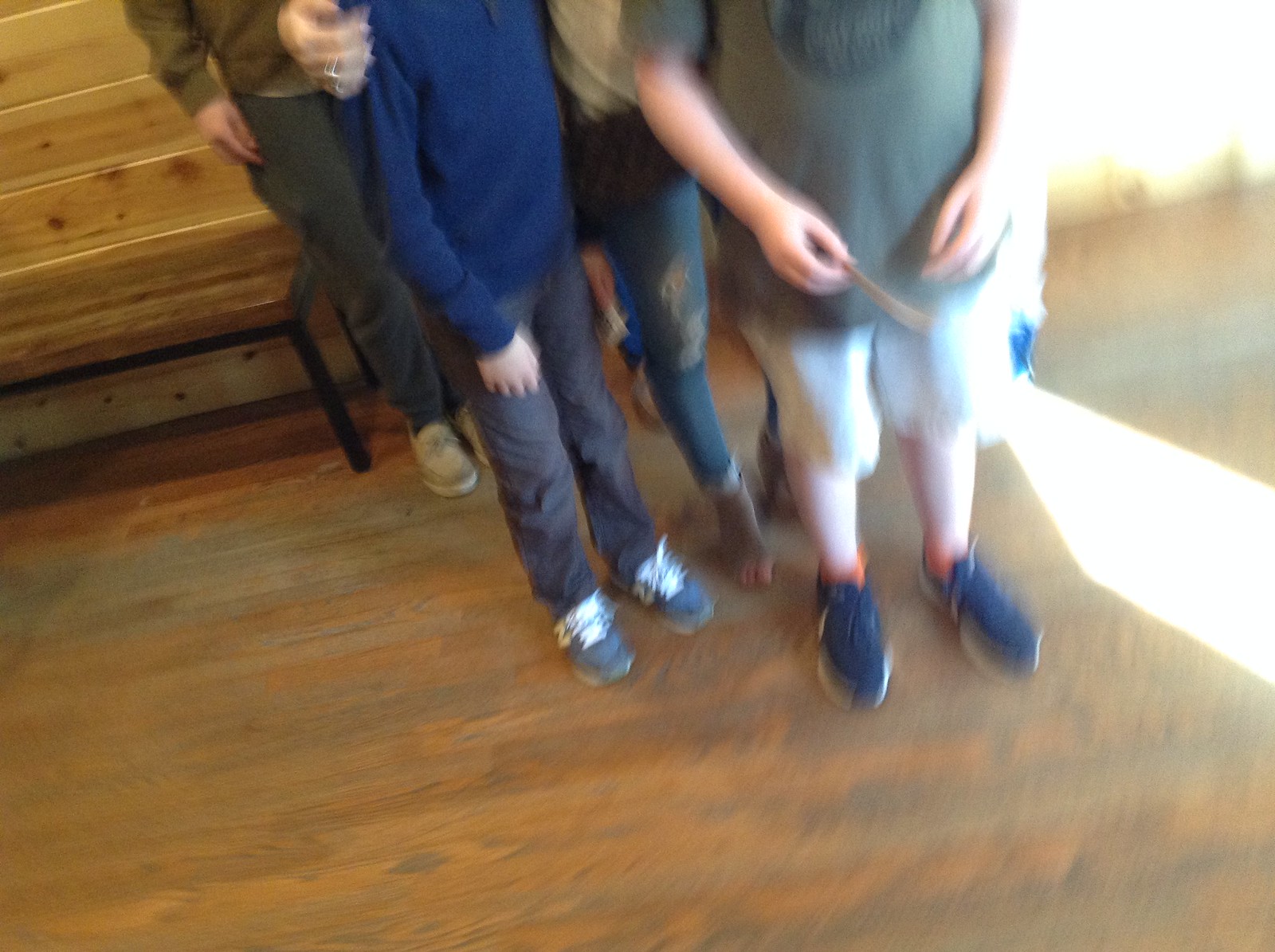A photograph captures a group of four individuals, but the camera angle points slightly downward, framing their torsos downwards and obscuring their shoulders, heads, and faces. To the right, a person is dressed in a t-shirt, shorts, and sneakers. Behind this individual stands a woman in skinny jeans with ripped knees, who is embracing a young boy clad in a blue jumper, jeans, and trainers. In the background, another figure can be partially seen, revealing only their legs, feet, and a fragment of an arm. The scene is set on a wooden floor, with noticeable blur and motion streaks, indicating the camera was in motion when the photo was taken, adding a dynamic, albeit blurry, effect to the image.